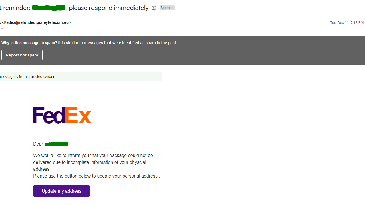This image is a very low-resolution screenshot of what appears to be the FedEx website. Key features observed include the FedEx logo, with "Fed" in dark purple and "Ex" in orange. At the top is a white bar containing text that is indecipherable due to the poor quality of the image. Directly below this is a charcoal gray bar, also containing text that is completely illegible. 

Beneath the gray bar, there is another line of text on a white background, which remains unreadable. The FedEx logo is prominently displayed again with a surrounding block of text, both of which are indecipherable. A purple button, matching the shade of "Fed" in the logo, is visible but its text cannot be made out. Interestingly, it appears that the screenshot has been edited to blot out certain parts of the text on the very top line and just below the FedEx logo, suggesting an intentional redaction, though the low resolution would have likely rendered this text unreadable regardless.